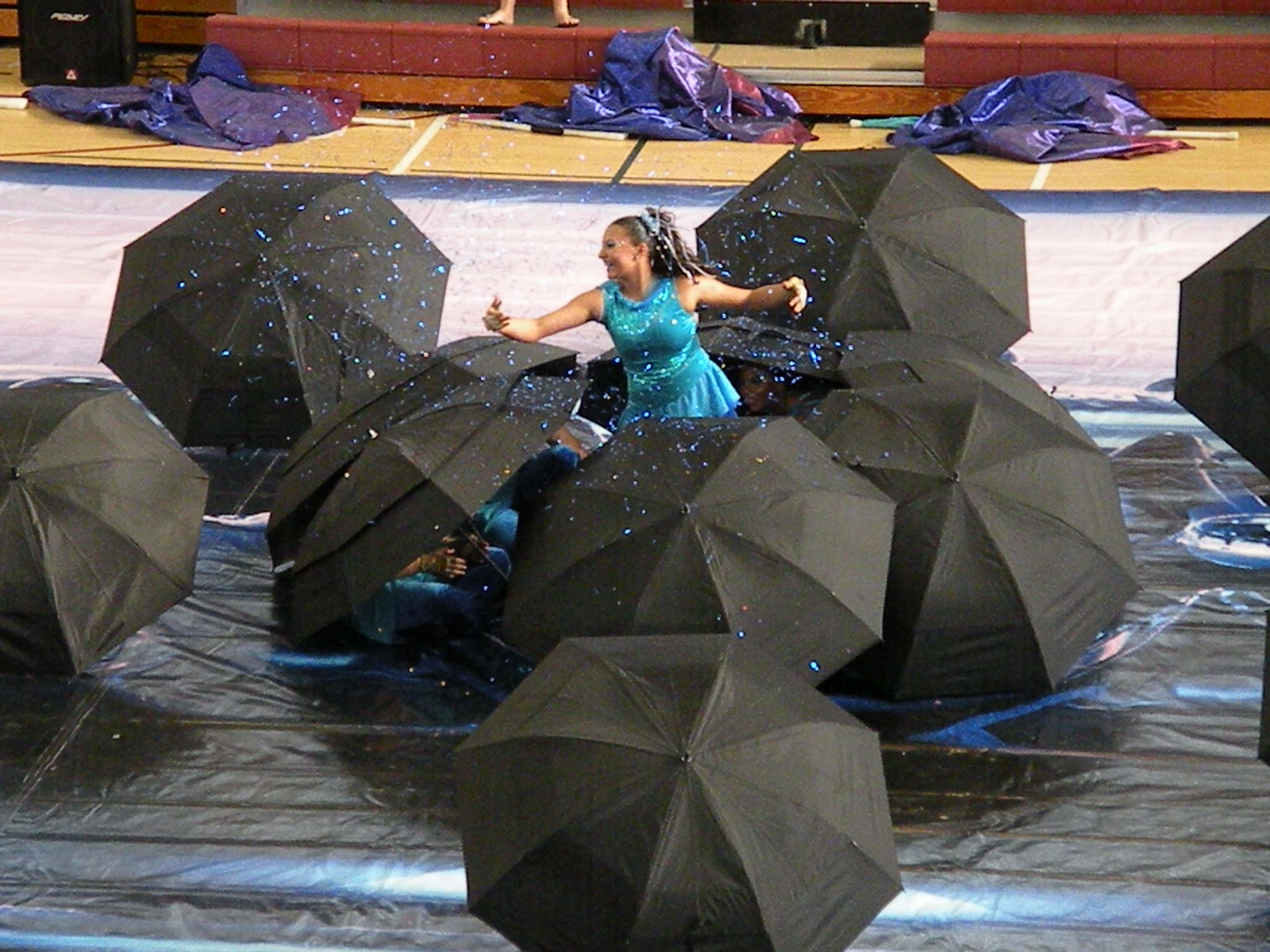In an indoor theater setting with light brown wooden flooring, an enchanting performance unfolds on stage. At the center of the photograph, a white-skinned woman dressed in a bright blue dress stands out vividly against a backdrop of falling confetti. She is smiling radiantly, with her arms spread wide, enveloped in the joy of the moment. Her black hair cascades down to her shoulders, adding to her striking presence. Around her, seated on the ground, a multitude of performers, also in bright blue dresses, peek out from beneath a sea of open black umbrellas, contributing to the scene's whimsical charm. The stage is adorned with three large pieces of purple fabric draped across the flooring, adding a touch of elegance. In the upper portion of the image, a pair of feet, white-skinned and belonging to another performer, dangle over the stage, adding a curious and playful element to the composition. A large black speaker sits prominently on the far left, further suggesting the vibrancy of the ongoing performance. The energy feels magical, as though the umbrellas and the confetti have transformed the stage into a poetic dreamscape.